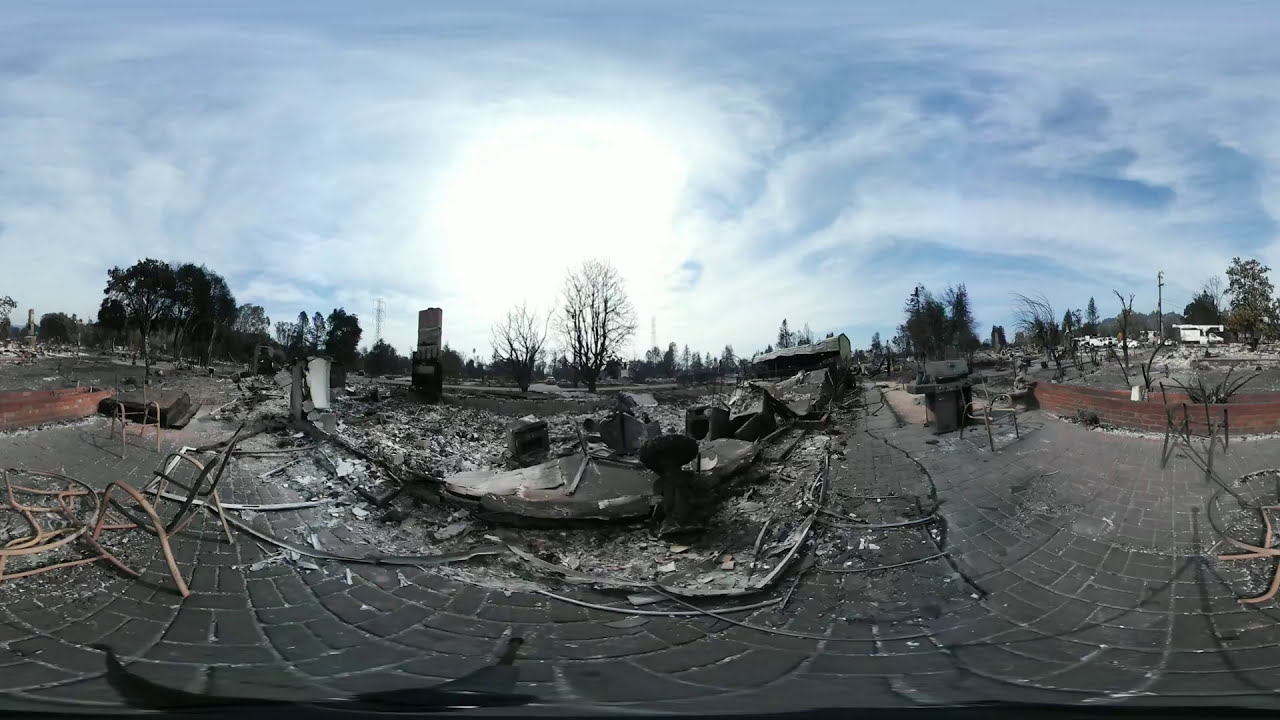The image is a detailed panorama of a scene depicting the charred remains of a burned-down structure, suggesting a devastating fire. The ground is strewn with broken pieces of cement, stone, and rubble, with twisted metal pipes and wires lying haphazardly. Amidst this destruction, remnants of what appears to be a building can be inferred from the considerable amount of debris and the general shape it forms.

On the left side of the image, there are frames of old chairs, while to the right, there is a gas grill with a metal chair in front of it, set against a small burned barn-like structure. The foreground features a brick patio, now dirtied with ash and soot. Behind this scene is a backdrop of trees and a few visible cars, indicating the presence of a road. The sky above is clear and blue, with the sun peeking out from behind some clouds, contrasting sharply with the somber situation below. The entire area, possibly an outdoor communal space or park, looks abandoned and bears the scars of an intense fire.